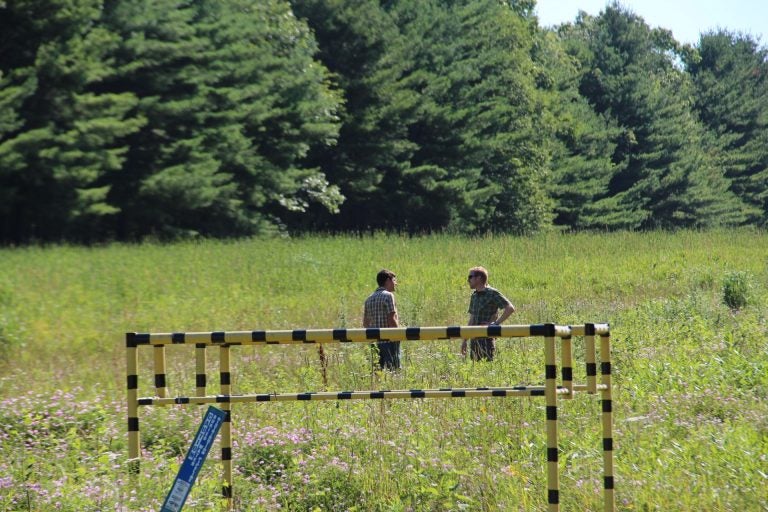In this detailed outdoor photo taken during the day, the landscape-oriented image captures a serene yet slightly overgrown scene. The upper portion of the photograph, accounting for about 40%, is dominated by enormous, lush green pine trees, slightly out of focus. Among them, the upper right-hand corner reveals a sliver of clear, bright blue sky. The lower 60% of the image features an expansive field with tall, unmowed grass, interspersed with patches of wildflowers, including noticeable spots of purple or pinkish blooms and a small bush.

Centrally located in the image, two young Caucasian men, both clad in button-down short-sleeved shirts and work pants, stand facing each other. Their legs are partially obscured by the tall grass, visible only from the knees up. The man on the right is in a darker shirt, while the man on the left is in a lighter one.

Prominently in the foreground stands a yellow-and-black-striped piping structure with four legs arranged in a rectangular formation from left to right. Additionally, a blue and white sign leans diagonally against one of the structure's legs, adding an industrial touch to the otherwise natural setting.